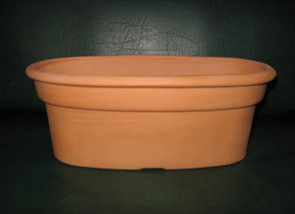The image is a small rectangular landscape photograph showcasing a terracotta-colored planter. This earthware planter, which may be either clay or plastic, features a thick rim at the top, tapering slightly towards the bottom. Its orangish-tan hue resembles that of typical outdoor flower pots. The planter is long and oval-shaped, reminiscent of a bathtub, with an empty interior that is only partially visible from the side angle depicted in the photo. It rests on a plain, dark surface, possibly a black table, with a black or dark gray wall directly behind it. The background is uniformly dark, except for a subtle light illuminating the planter and the wall above it, ensuring all focus remains on the pot. The detailed simplicity of the composition emphasizes the planter's structure and texture.